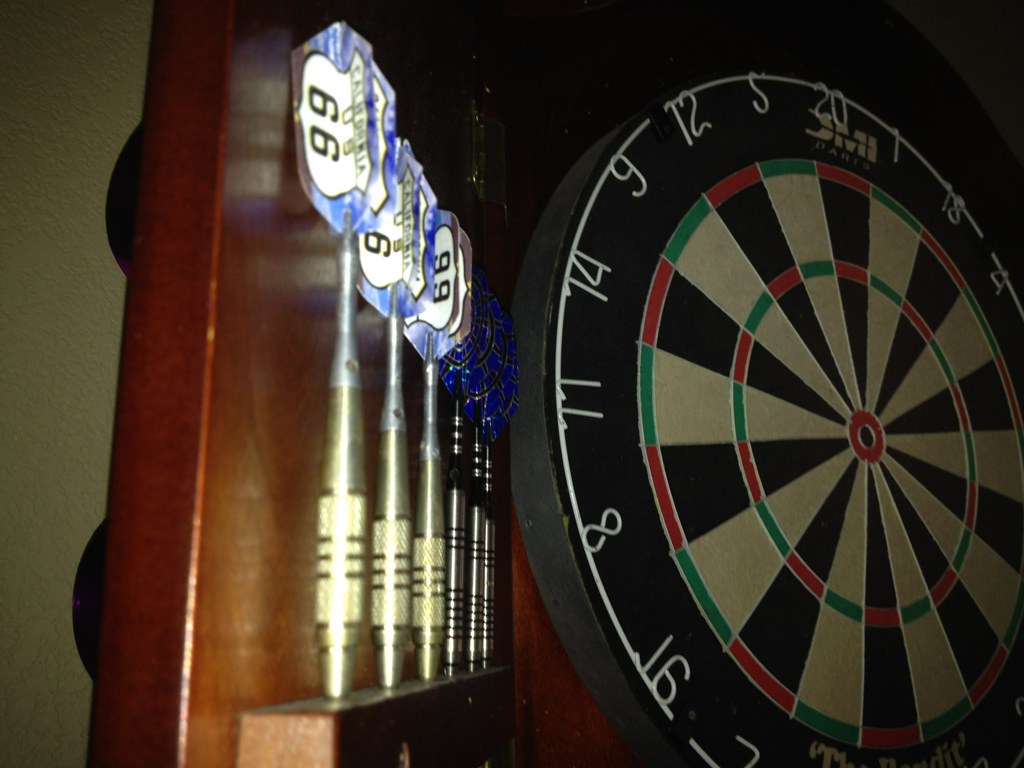In this detailed image of a dart setup, we observe a close-up shot of a dartboard accompanied by six darts housed within the open left door of a wooden dartboard cabinet. The dartboard itself, slightly dim compared to the brightly lit darts, displays numbers ranging from 8 to 14 around its black face. This face is segmented into concentric rings of alternating colors: black, red, green, tan, with a vivid red bullseye in the center.

The darts, with high-quality silver barrels, stand upright in their holder affixed to the inside of the left cupboard door. These darts are detailed with white-background labels on their blue fins, displaying text such as "Route 66" and "California 66." The door is positioned at an angle, giving a side view that highlights three rows of darts. The backdrop, made of wood and visibly brown, complements the dark-toned dartboard, which features brand markings possibly indicating "SMI."

Despite the overall darkness of the image, the contrast between the gleaming darts and the subtler tones of the dartboard provides a rich visual depth, enhanced by the meticulous arrangement of the darts in their holder. This setting implies a readiness for a potential dart tournament, with its precise assembly and high-quality equipment emphasizing the competitive spirit.